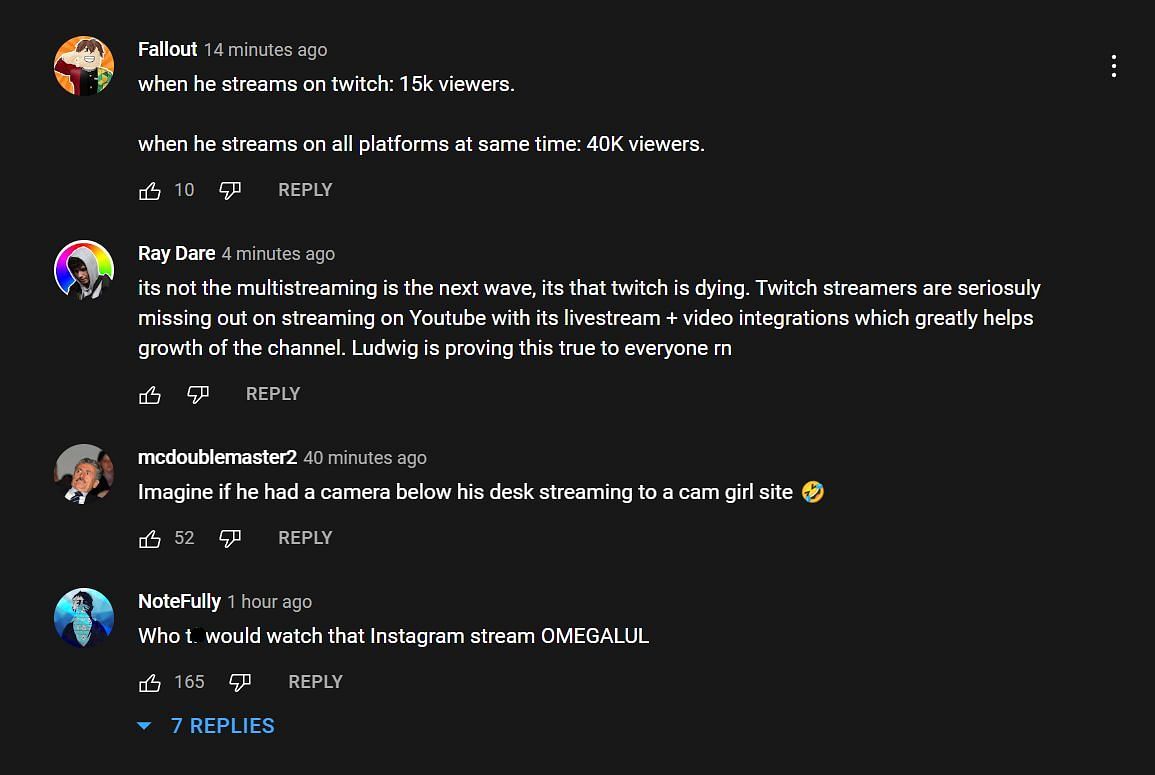This is a detailed screenshot of the YouTube comment section in dark mode, where the background is black. The comments pertain to streaming platforms, comparing viewership and advantages.

1. **User:** Fallout  
   **Posted:** 14 minutes ago  
   **Comment:** "When he streams on Twitch, 15,000 viewers. When he streams on all platforms at the same time, 40,000 viewers."  
   **Engagement:** 10 likes  
   **Profile Picture:** Likely a Lego or Roblox avatar  
   **Additional Info:** There's an option to reply to the comment, but dislikes are not displayed.

2. **User:** Ray Dare  
   **Posted:** 4 minutes ago  
   **Comment:** "It's not that multi-streaming is the next wave; it's that Twitch is dying. Twitch streamers are seriously missing out on streaming on YouTube with this live stream plus video integration, which actually helps grow the channel. Ludwig is proving this true to everyone right now."  
   **Engagement:** No likes or dislikes  
   **Profile Picture:** Depicts a person in a hoodie looking down.

3. **User:** McDoubleMaster2  
   **Posted:** 40 minutes ago  
   **Comment:** "Imagine if he had a camera below his desk streaming to a camgirl site 😂."  
   **Engagement:** 52 likes  
   **Profile Picture:** An older man leaning back in a chair, dressed in a suit and tie.

4. **User:** NoteFully  
   **Posted:** One hour ago  
   **Comment:** "Who [crossed out] would watch that Instagram stream OmegaLul."  
   **Engagement:** 165 likes, 7 replies (not shown)